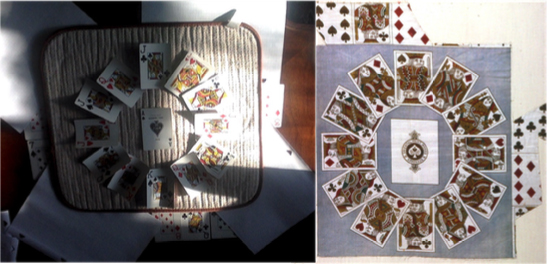The image is a side-by-side comparison of two photographs. 

**Left Side:**
The left photograph appears to feature a dark wooden table, although it could possibly be the floor; it's difficult to discern due to the image quality. Scattered across the table are some indistinct objects, possibly pieces of paper, though their exact nature is unclear. Sunlight streams in from a nearby window, casting bright spots and shadows that add to the ambiguity. In the center of the setup is a square mat, resembling a kitchen drying mat. Arranged in a circular pattern on this mat are playing cards from a standard deck. One card sits in the middle of the circle, while additional cards are partly tucked beneath the edges of the mat on three sides.

**Right Side:**
The right photograph shows a similar arrangement but with clearer detailing. The playing cards are again placed in a circle with one card in the middle. These cards rest on a gray square fabric, which itself is situated on a table. Beneath this gray fabric is another layer of fabric featuring decorative designs, adding an extra layer of texture and intricacy to the setup.

Both photographs seem to capture a unique and somewhat perplexing arrangement of playing cards, providing an intriguing visual comparison.